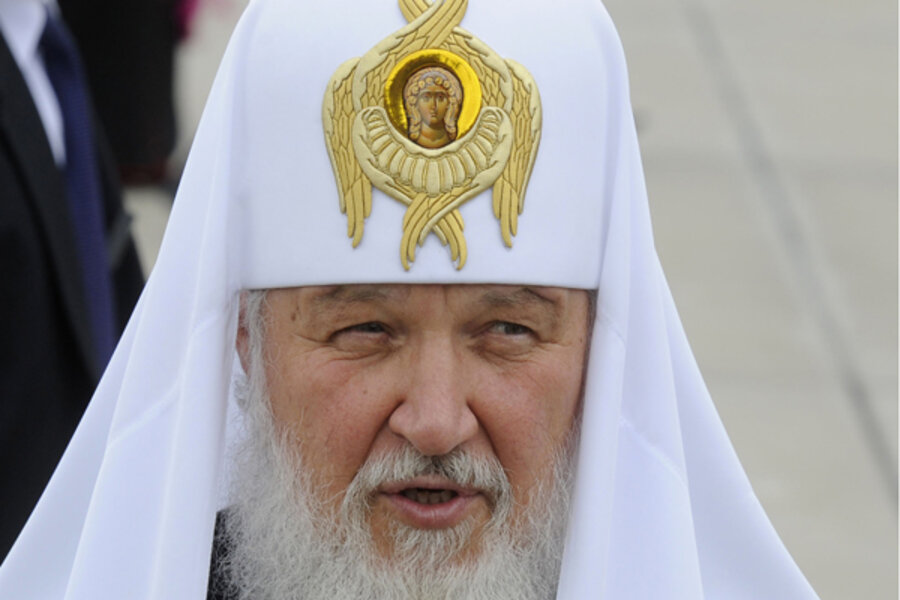This photograph features an older man with a prominent grey beard and mustache, suggesting a religious figure, possibly a priest. He wears a white cap adorned with a golden design of interlocking wings and a central circular emblem depicting a significant religious figure, potentially Jesus or Mother Mary. The man appears to be speaking, facing slightly to his left, which is the right side of the photograph. The background is blurred but shows other people, including a person in a black suit, white dress shirt, and blue tie or lanyard. The image lacks any identifying information regarding the name or location.